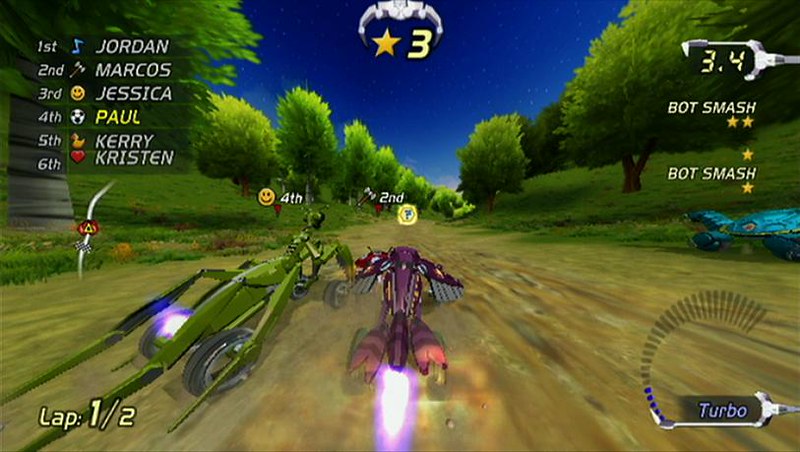The image features a vibrant screenshot from a video game, showcasing an exhilarating motorcycle race. Dominating the scene are two distinct motorcycles: a large green one ridden by a green skeleton, and a purple one emitting impressive flames from its rear, piloted by a purple character. The race unfolds on a rugged dirt road, set against a scenic backdrop of rolling green hills, lush grass, and abundant trees under a clear blue sky. A boardwalk climbs the side of one of the hills, adding to the picturesque landscape.

Displayed on the screen are game statistics and player information. At the top, "Lap 1 of 2" and "Turbo" are indicated, suggesting the players are in the midst of a competitive match. To the side, white numbers read "3.4" and "Bot Smash," clearly marking progress and objectives within the game. The player rankings listed include Jordan, Marcos, Jessica, Paul, Carrie, and Kristen, showcasing a lively and competitive gaming experience.